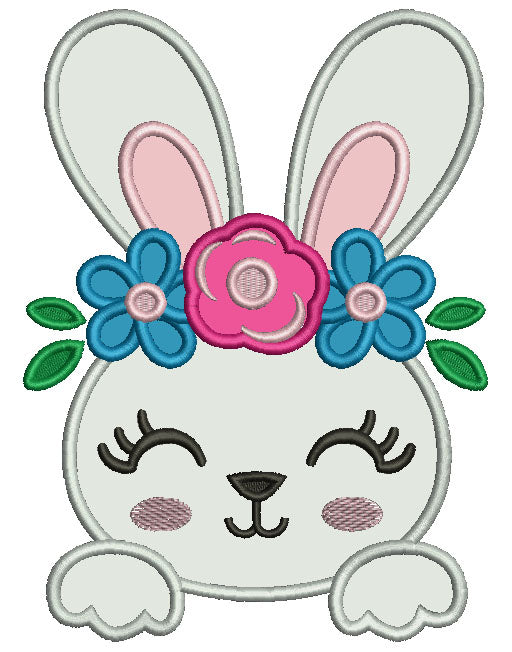The image depicts an embroidered applique patch featuring a cute, cartoony white bunny. The bunny's head and ears are prominent, with the front paws positioned below its cheerful face. The bunny has large white ears with small pink semi-circular shapes at the lower part of each ear. Its face is an oval shape, adorned with closed eyes represented by black arches and long black eyelashes. The bunny's cheeks are highlighted with pink ovals, and its nose is depicted as a small black half-circle with two hooks. On top of the bunny's head rests a vibrant floral headdress, consisting of a bright pink flower in the center and two blue flowers on either side. Each flower includes pink and pinkish-white bulbs, complemented by two green leaves extending from the sides. The overall design of the patch is charming and whimsical, ideal for adding a touch of cuteness to any clothing item.